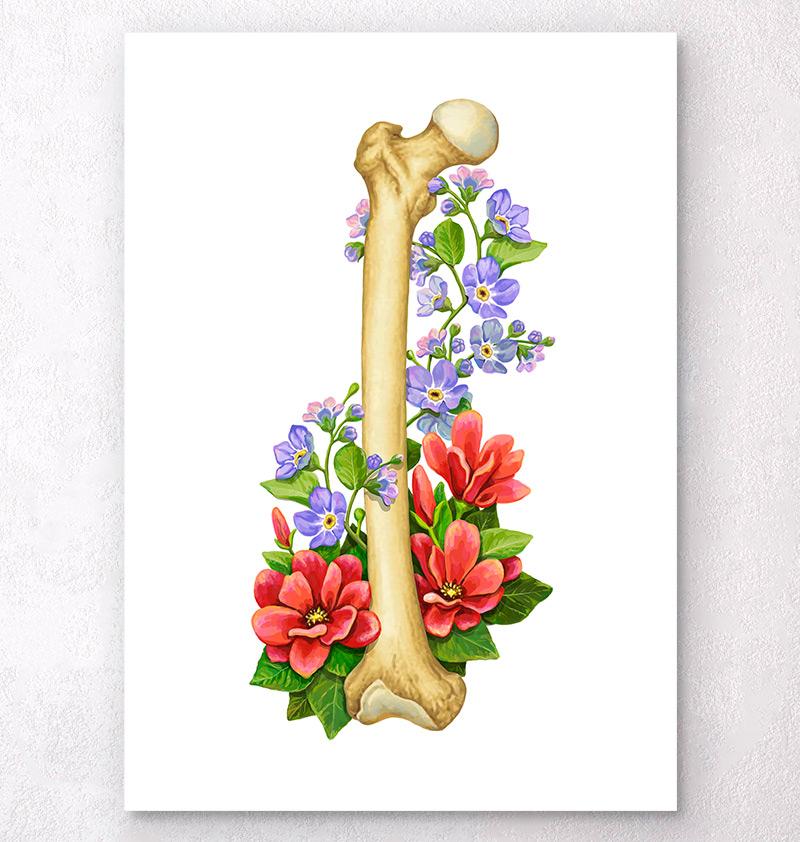The image depicts a captivating painting of a human thigh bone, shown against a plain gray wall. The bone, yellowish-white in color, is oriented vertically on a white, rectangular canvas. The anatomical detail includes a rounded bottom and a ball joint at the top, suggesting it is the femur, connecting to the hip. Adorning the bone are various vibrant flowers: large red-petaled flowers with yellow centers at the base, winding upward to reveal smaller purple flowers with yellow centers and even petite pink flowers towards the top. The flowers are nestled among green leaves and delicate stems, forming a striking contrast with the bone and creating an intricate blend of nature and anatomy.